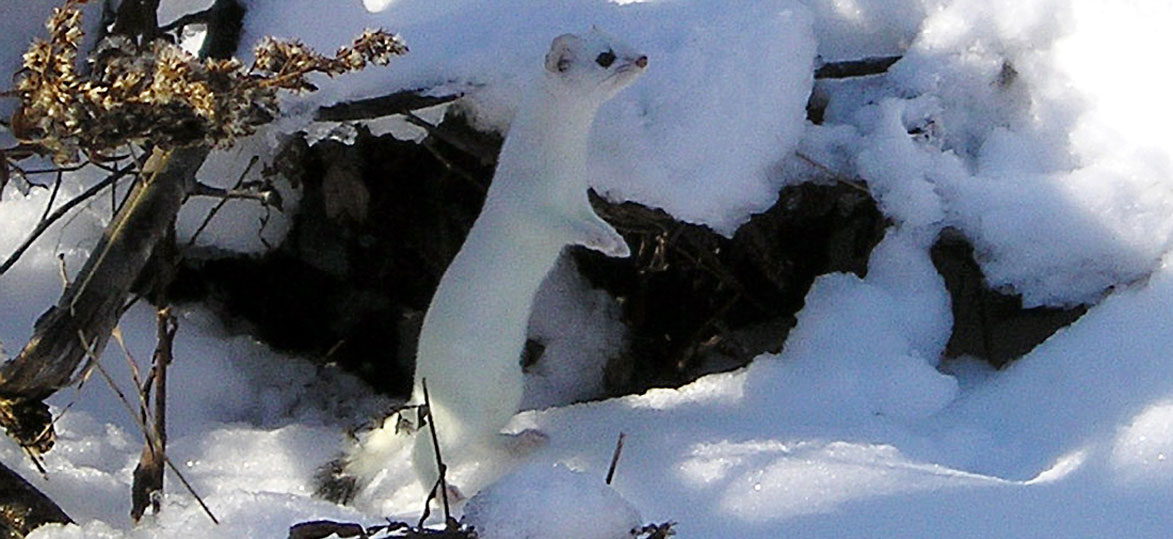In this detailed photograph, we see a white ermine, a slender-bodied mammal with white fur, standing attentively on its hind legs amidst a snowy landscape. The ermine, captured in a side profile, has small black eyes and long black whiskers, blending seamlessly into the predominantly white surroundings. The animal's little front legs are held out as it gazes to the side, with light filtering through trees or bushes in the background, illuminating the scene. The snow bank in which the ermine stands is mostly pristine and fluffy, save for some partially melted patches and scattered debris such as sticks. To the left of the image, a tree branch with a dried leaf is visible, adding an extra touch of detail to the natural scene. The photo is zoomed in, offering a clear and focused view of the ermine while encapsulating the serene and slightly varied snowy terrain in the background.